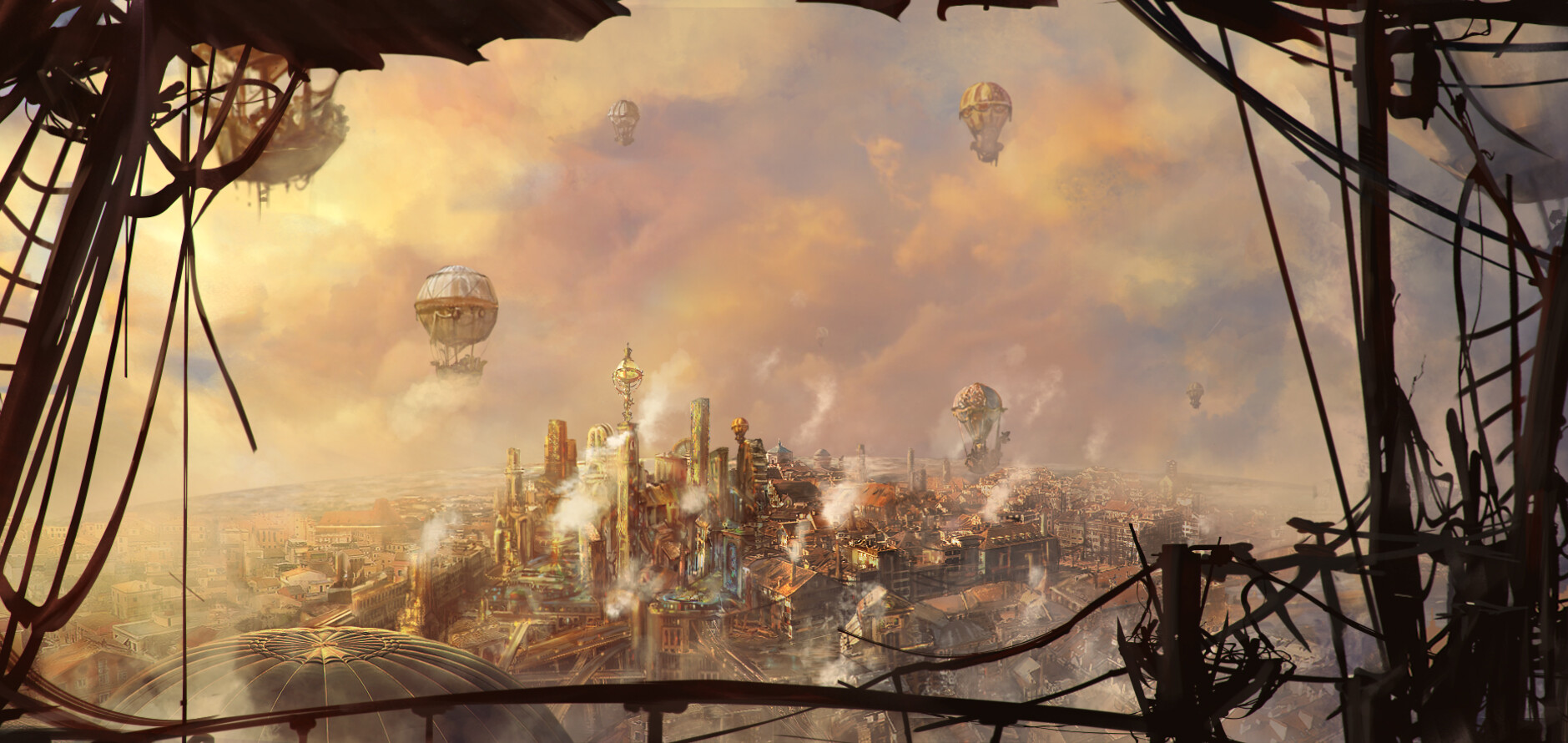A panoramic scene, possibly an oil or acrylic painting or from a video game, depicts a dreamy cityscape as viewed from a hot air balloon. The background, painted with a soft-focus technique, features a heavily clouded sky with the sun shining through from the upper left, casting hues of oranges and purples. Multiple hot air balloons, around five or six, dot the sky at varying distances, with a particular one almost directly below in the lower-left corner. The viewpoint includes the brown ropes and ties of the hot air balloon the viewer is in, along with the cables that likely anchored it. Below, the city unfolds with predominantly gold and brown-toned buildings mingling with wispy clouds or smoke, creating an ethereal atmosphere. The overall scene blends a light blue sky with purplish and bluish clouds, enhancing the enchanting and whimsical quality of the image.